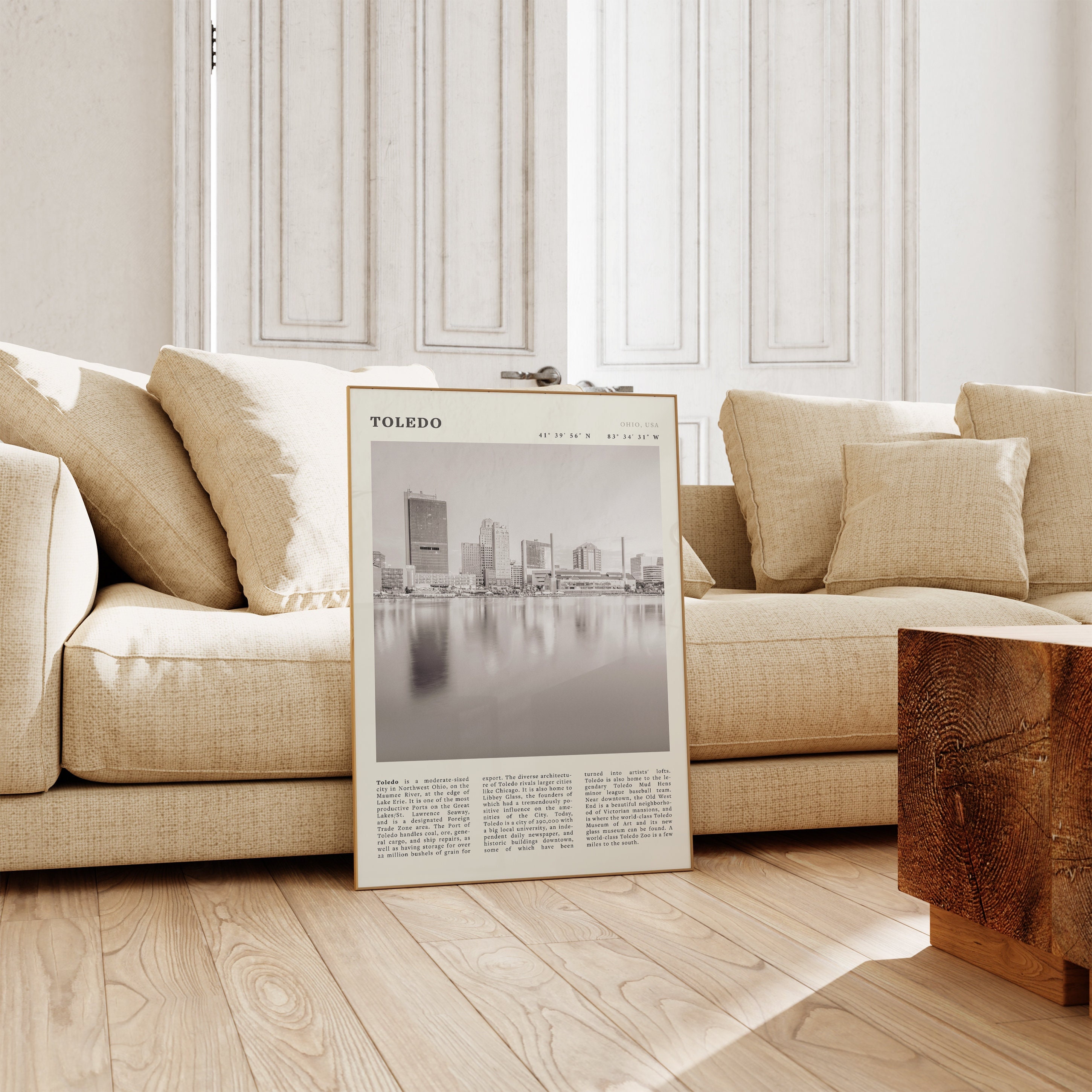The image depicts a serene lounge with off-white walls and a wooden floor. Dominating the background are large, white-painted double doors with metallic handles. In front of these doors stands a modern, square-shaped beige couch made of canvas fabric and adorned with six square cushions. Centered on the couch is a large framed black and white photograph featuring the skyline of Toledo, Ohio. This photograph prominently displays the title "Toledo" at the top, followed by "Ohio USA" alongside longitude and latitude coordinates in the top right corner. Below the image, three columns of text provide details about Toledo, stating it is a moderate-sized city in Northwest Ohio. The room is well-lit with beautiful natural sunlight streaming in from the side, adding to the cozy atmosphere. Completing the setting, a substantial wooden block coffee table is positioned on the wooden floor in front of the couch, maintaining a harmonious balance with the brown tones throughout the room.